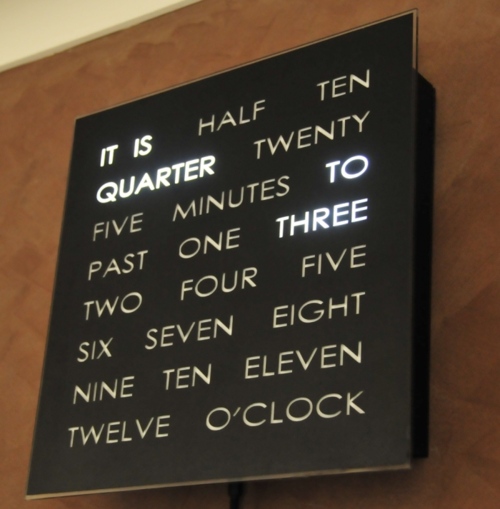The image features a stylish black frame or plaque mounted on a wall. The background of the frame is also black, creating a sleek and modern appearance. White text is displayed on the plaque, with some words illuminated to indicate the current time. The text includes phrases such as "half 10," "quarter 20," "five minutes to/past," and numbers from 1 to 12 followed by "o'clock." This unique timepiece functions as a visual clock, designed to help users tell time using words rather than traditional numbers.

In the current display, the illuminated text reads: "It is quarter to 3." This setup is extremely user-friendly, making it easy to read the time without needing to interpret numbers. The clock combines functionality with aesthetic appeal, offering a fashionable and visually pleasing addition to any space.